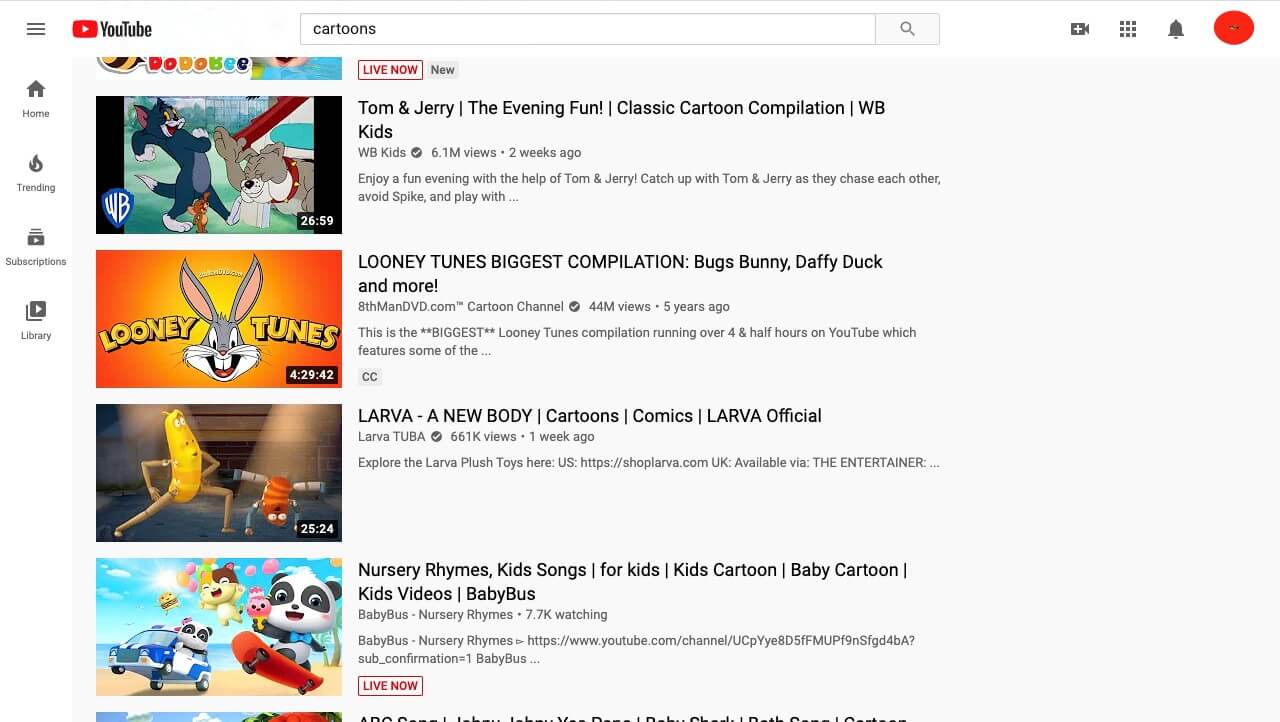This image depicts a YouTube webpage featuring a search for cartoons. In the upper left corner, the interface includes a stacked, horizontal, three-line "hamburger" menu icon. Next to it, the YouTube logo is displayed prominently, featuring bold black text and the iconic red rectangle with a white play button arrow inside. Below the search bar are four thumbnail images, each representing different cartoon videos.

1. The first video thumbnail displays characters from Warner Bros., specifically Tom and Jerry, alongside a gray bulldog. The video’s timestamp reads 26:59. To the right of the thumbnail, the title and description indicate it's a "Tom and Jerry: The Evening Fun - Classic Cartoon Compilation WB Kids."

2. The second video features a large image of Bugs Bunny, denoting it as a Looney Tunes cartoon.

3. and 4. The next two thumbnails feature additional cartoon videos aimed at kids, each accompanied by brief descriptions.

The layout is designed to help users quickly find and access entertaining cartoon content for children.